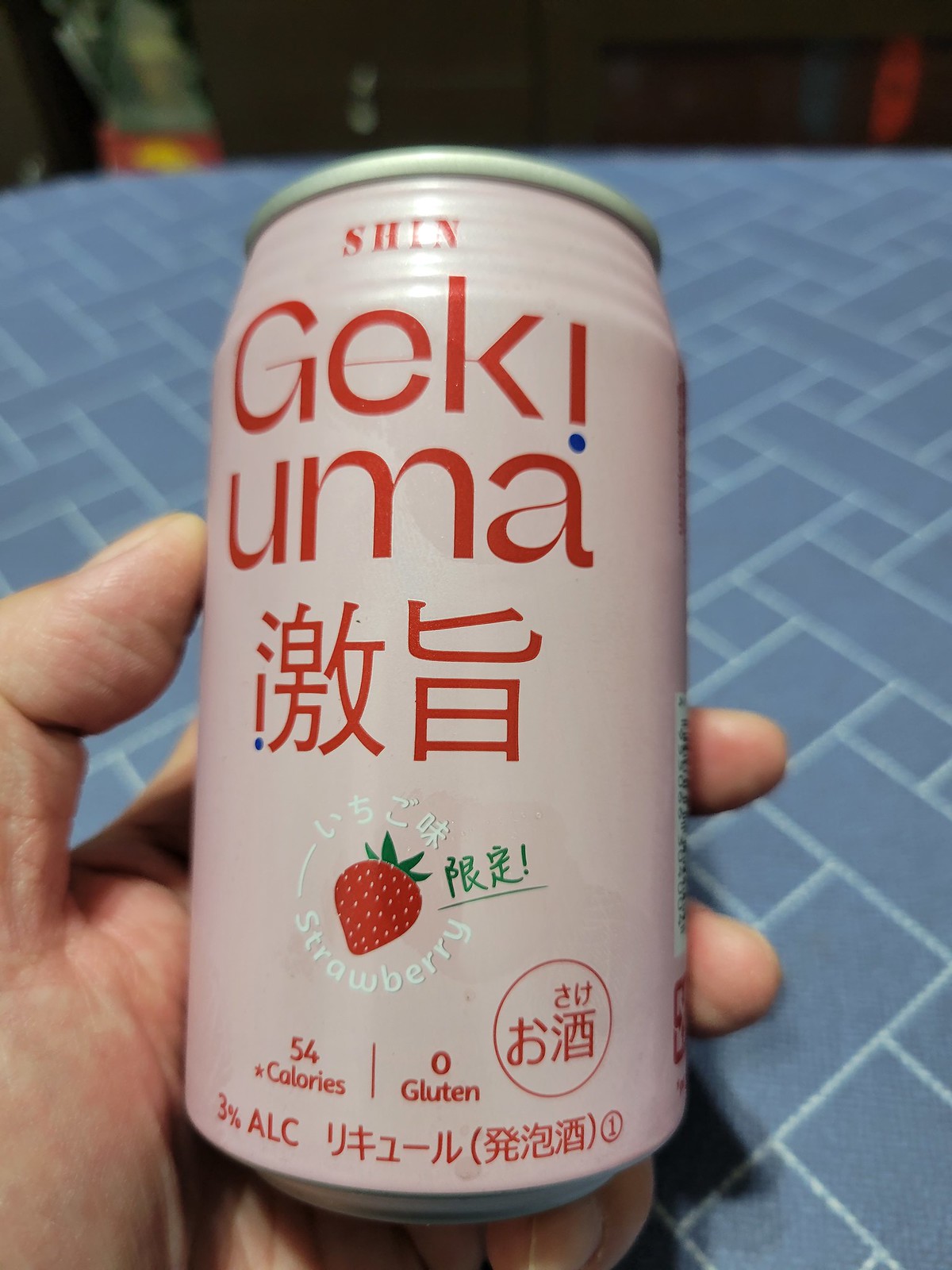In this vertically rectangular indoor photo, a light blue tablecloth with intersecting white lines creating squares and rectangles serves as the background. From the lower left corner, a portion of a left hand is visible, with the thumb extending upwards and slightly outwards. The hand is grasping a beverage can with a very pale pink base color and red lettering. The top of the can features the text "Shin Geki Uma." Beneath this, there are two symbols, possibly Japanese or Chinese. Further down, a red illustration of a strawberry appears, with the word "strawberry" written in a curved white font underneath. Additional details on the can include "54 calories, zero gluten" printed in red, followed by "3% alcohol" and more Japanese or Chinese symbols below.